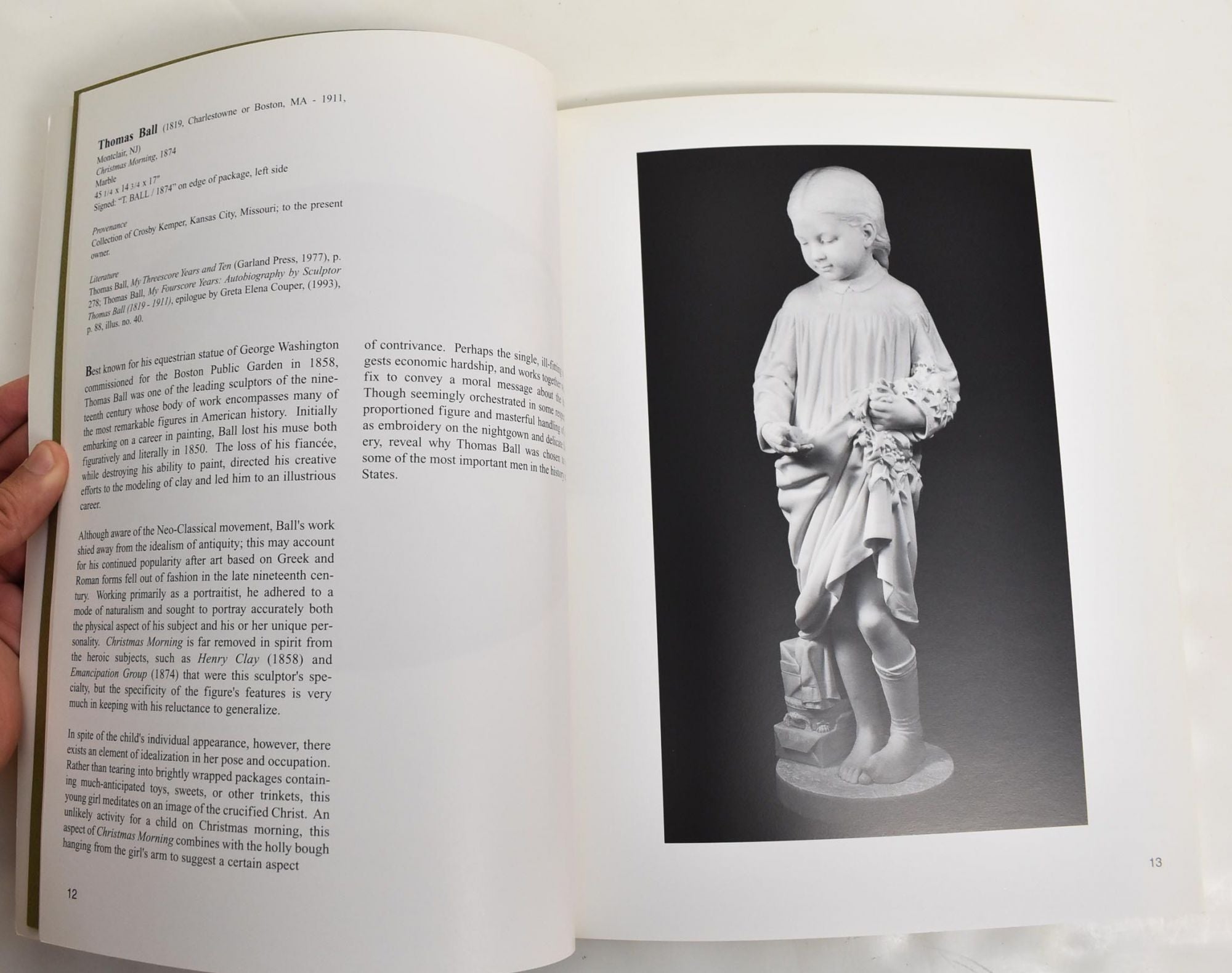The photograph depicts a person holding open a book to two specific pages. The right-hand page, labeled as page 13, features a full-page black-and-white image of a marble statue of a young girl, probably around 10 years old, from a different era. The girl is depicted in a detailed nighttime outfit, resembling a gown or pajamas, with socks pulled above her ankles. The girl, with her hair pulled back, is holding up the bottom of her gown to expose her knee, where one sock appears. She stands on a small rug, beside a couple of bags. The left-hand page, marked as page 12, contains a description centered around the sculptor Thomas Ball, mentioning his well-known equestrian statue of George Washington commissioned for the Boston Public Garden in 1858. The text extends into a detailed biography of Ball, highlighting his transition from painting to sculpture after the loss of his muse in 1850, and his subsequent rise as a leading sculptor of the 19th century. This biographical text spans three paragraphs, diving into his artistic journey and notable works.